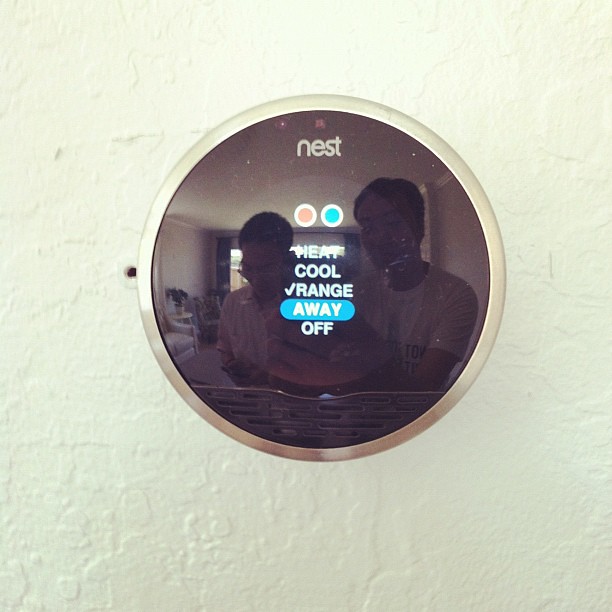In the image, we see a circular smart home thermostat, specifically a Nest device, seamlessly integrated into the wall. The thermostat features a highly reflective black glass touchscreen, bordered by a sleek stainless steel silver trim. The screen displays various settings, including options for "Heat," "Cool," "Range," "Away," and "Off." Reflecting off the glossy surface of the device, the living room in which it is installed is visible, along with the faint image of two men capturing the photo with a smartphone. The top of the screen prominently displays the "Nest" branding, indicating the manufacturer.